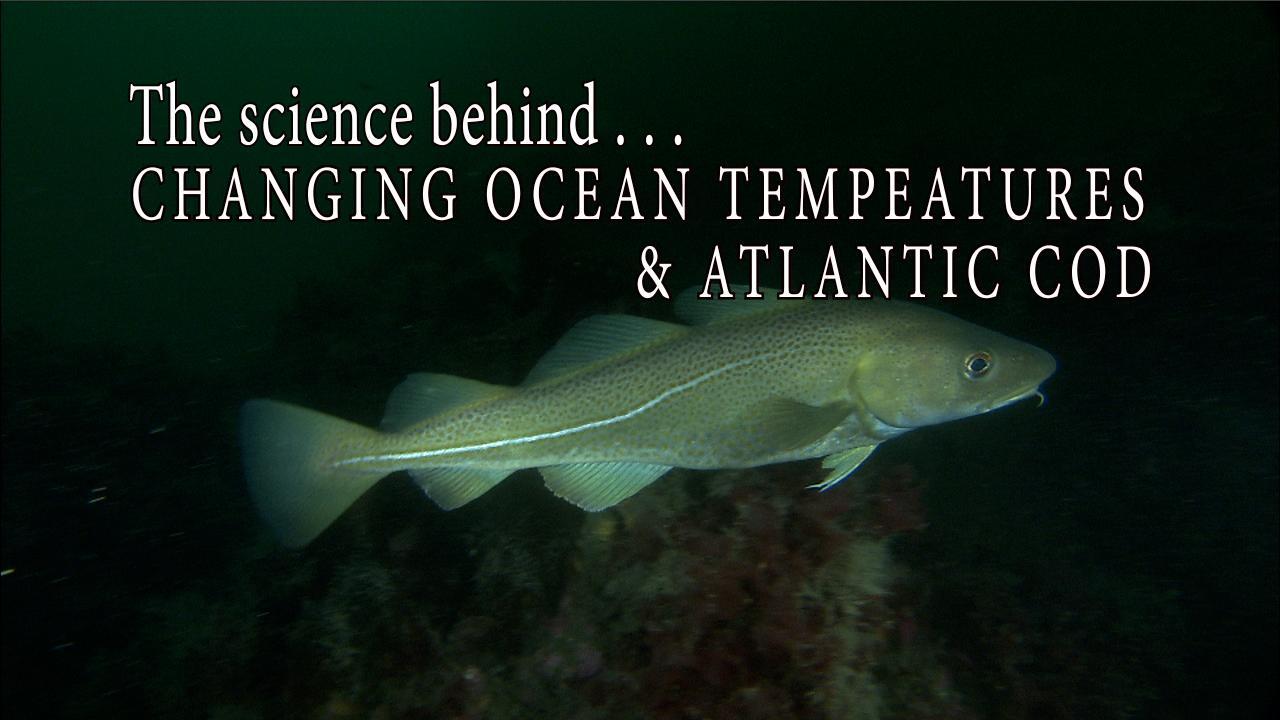The image features a greenish Atlantic cod swimming in dark, underwater surroundings, suggesting deep ocean depths. The background is black, enhancing the visibility of the fish and its features. The fish faces right, displaying a white stripe that runs from just behind its gills almost to its tail. It has three fins on top, two fins on the bottom, and a small additional fin near the front. Below the fish lies a large, light green and brown stone, perhaps indicating the ocean floor. The text above the fish, written in white, reads "The Science Behind... Changing Ocean Temperatures and Atlantic Cod," though there's a typo in the word "temperatures." The title has "The Science Behind" in lowercase except for the capital 'T', while the rest of the words are capitalized. The fish's eye is distinctly visible, complementing its overall detailed depiction against the dark water backdrop.